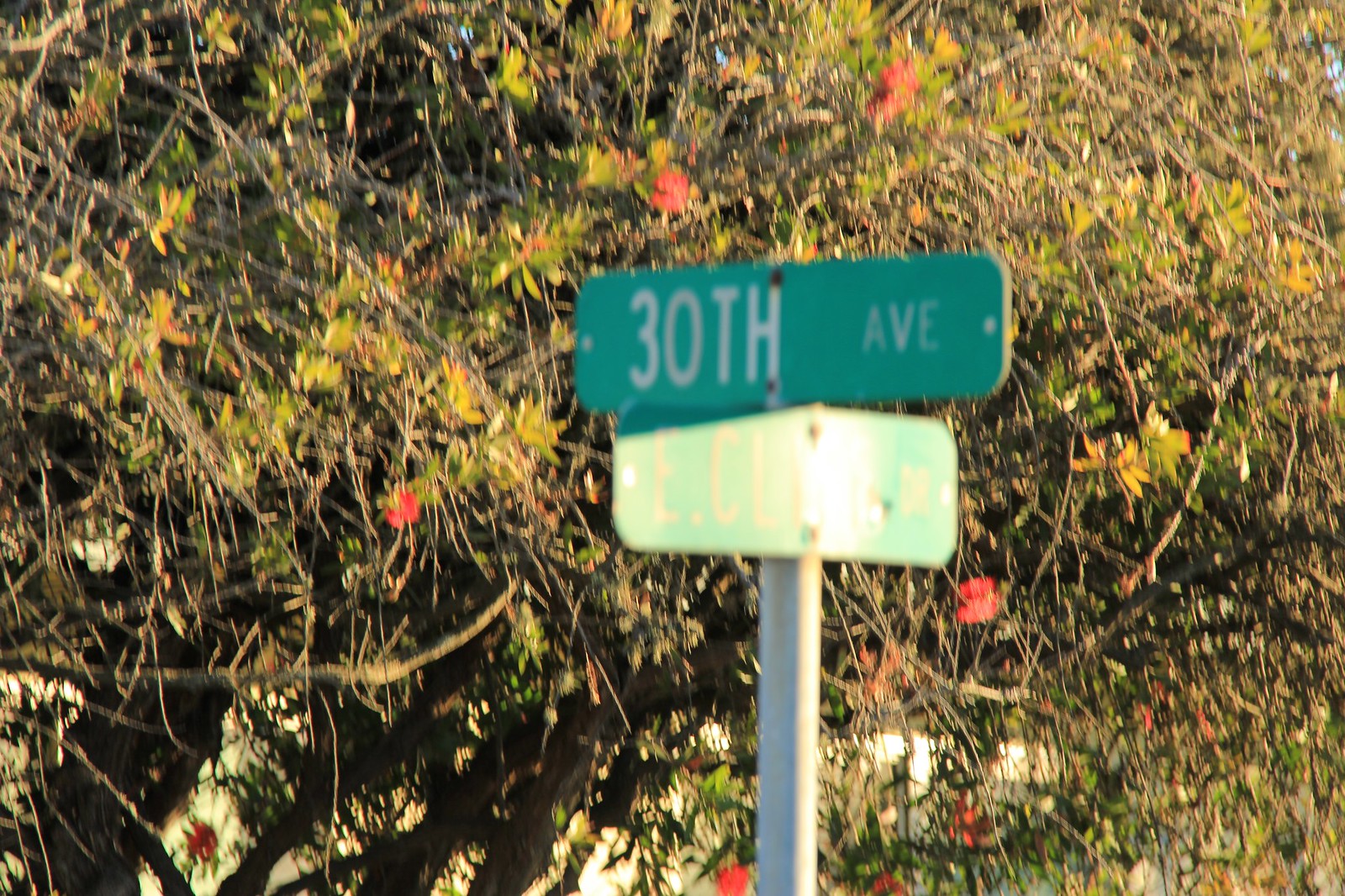The image is a first-person POV shot centered on a sign attached to a white post. The main sign, which is green with white lettering, reads "30th Ave," indicating "30th Avenue." Positioned directly below this is another sign, angled in a criss-cross manner from right to left rather than horizontally. This secondary sign appears almost yellow due to the intense glare of the sun, making it difficult to discern any writing on it; however, it might also be green with the lettering obscured by the sunlight. In the background, there is lush foliage from trees, with glimpses of blue sky seen through the leaves at the top of the image.